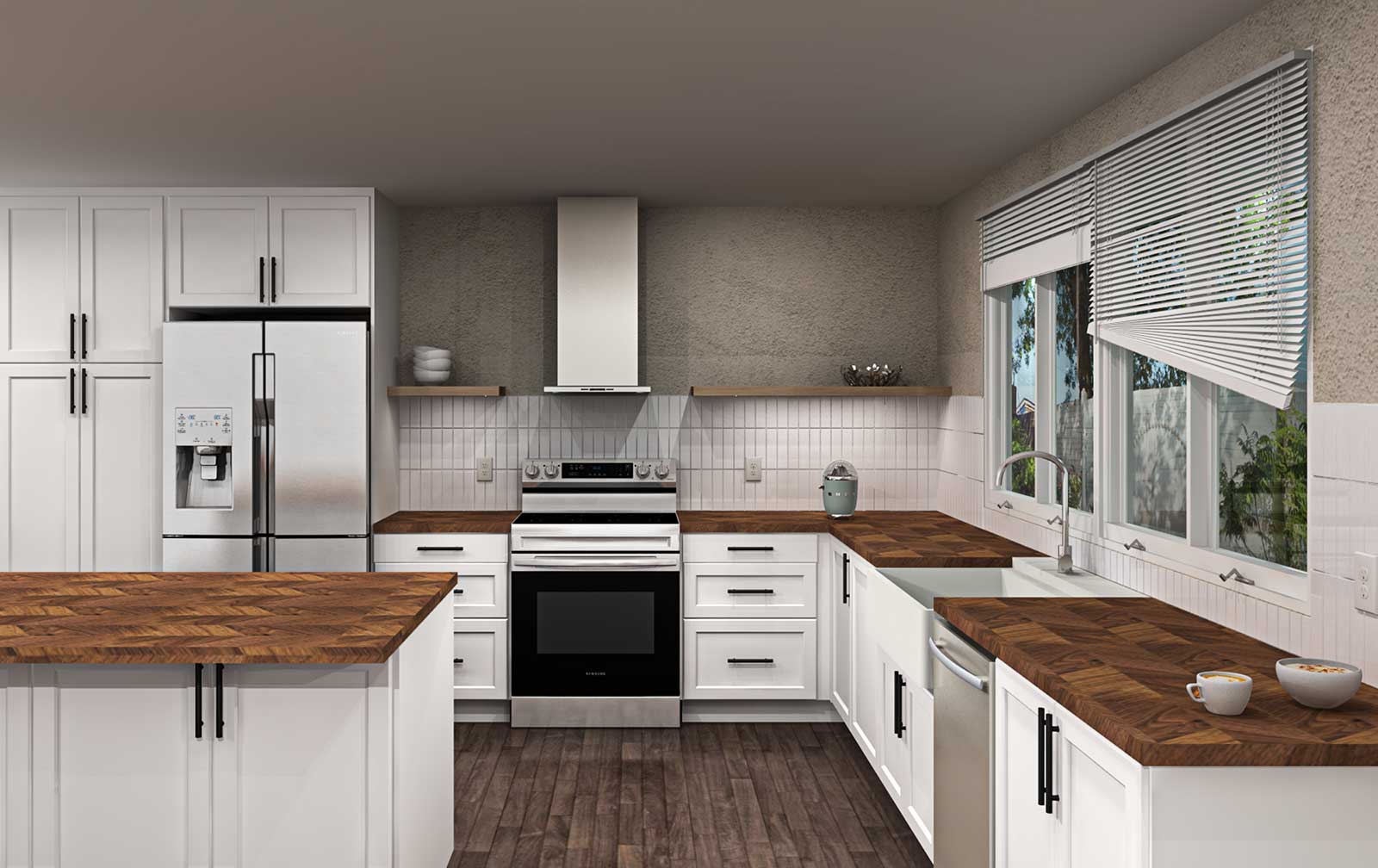This is a detailed photograph of a modern kitchen with muted colors. The kitchen features white cabinets adorned with long, slim black handles, some of which are hanging slightly crooked. The countertops are a dark brown butcher block with a parquet-like texture. On the left side, there is a white refrigerator next to a tall cabinet, and above the refrigerator, there is a small cabinet. Central to the kitchen is an electric stove flanked by cabinets with multiple drawers. Adjacent to the stove, there is open shelving and stainless steel appliances.

The right side of the kitchen showcases a sink situated under a series of large windows, some with Venetian blinds that are either fully raised, crooked, or halfway down, revealing a view of greenery outside. The floor is covered with brown wooden planks, complementing the dark countertops. Additionally, there is a kitchen island on the left side with more cabinetry. Notably, a cup and a bowl can be seen on the edge of the countertop on the right, near the sink.